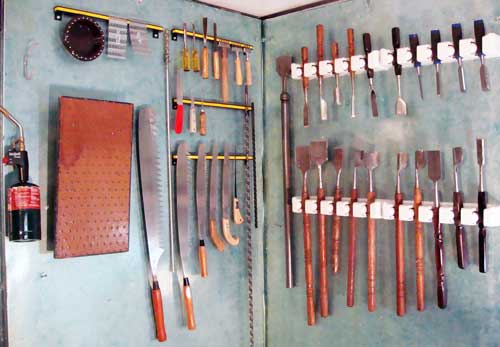The image depicts a highly organized woodworking shop, showcasing both walls of a corner. Each wall is covered in sleek, silver metal panels and features a variety of tool organizers. On the right wall, there's a comprehensive array of woodworking chisels displayed on two long racks, each chisel varying in width and length. The left wall hosts a more eclectic collection of tools, including six or seven different-sized saws hanging from yellow rods and an older piece of pegboard for additional storage options. A propane-fueled handheld blowtorch is also hanging on this side. Further detailing includes a long saw with a wooden handle, numerous files, and an iron bar with a knurled end. There's even what appears to be a brass bar with hanging items, possibly paper, contributing to the meticulous arrangement. Overall, this well-stocked workshop corner reflects a woodworker's dedication to maintaining a well-organized array of hand tools.